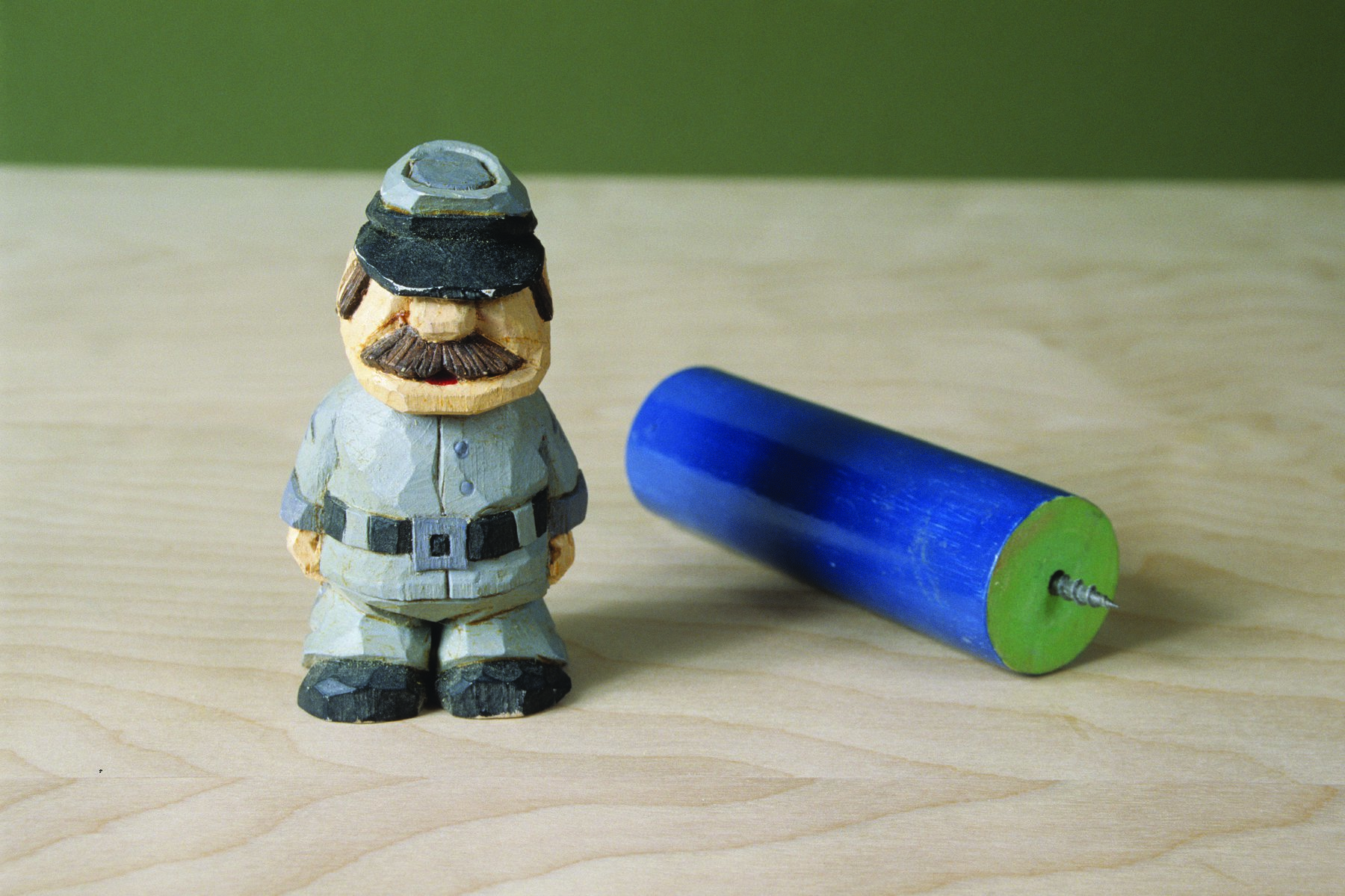In this image, there is a finely detailed hand-carved wooden figurine of a man, reminiscent of a Civil War soldier. The figure is adorned in a grey uniform with a matching hat that has a black brim. His footwear is consistently noted as black shoes. Prominent facial features include long sideburns, a big nose, and a bushy brown mustache. His eyes are obscured under the brim of his hat. The soldier stands upright on a wooden table, next to a small blue dowel or cylinder. This cylindrical object is painted blue with green ends and has a small metal screw protruding from one end. The surroundings outside of the table have a greenish hue, but the primary focus remains on the wooden soldier and the curious dowel beside him. The overall color palette includes shades of blue, green, grey, black, tan, and flesh tones.